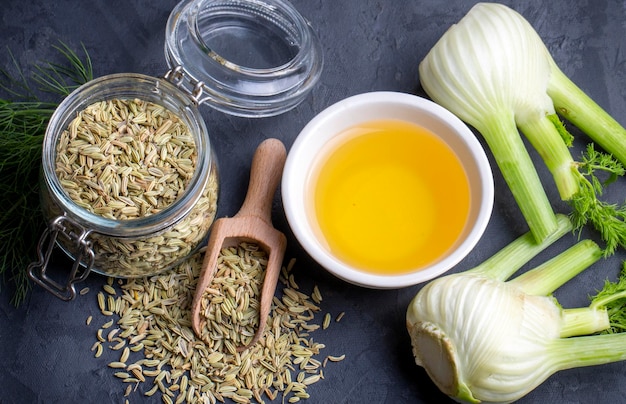In this color photograph, a rustic food arrangement is displayed on a blue tablecloth. Central to the composition is a white bowl filled with a vibrant yellow liquid, possibly oil or broken yolk. This bowl is surrounded by an array of fresh vegetables, predominantly leeks with their white bulbs and green stems, positioned to the right. To the far left, a wooden scoop containing seeds rests on the tablecloth, alongside a clear glass jar with a metal clasp. The jar is filled with more seeds, some of which have spilled out onto the fabric. Behind the jar, green leaves, perhaps herbs, add an additional touch of freshness to the scene. The background is a neutral, black color, drawing focus to the vibrant and textured food display in the foreground.